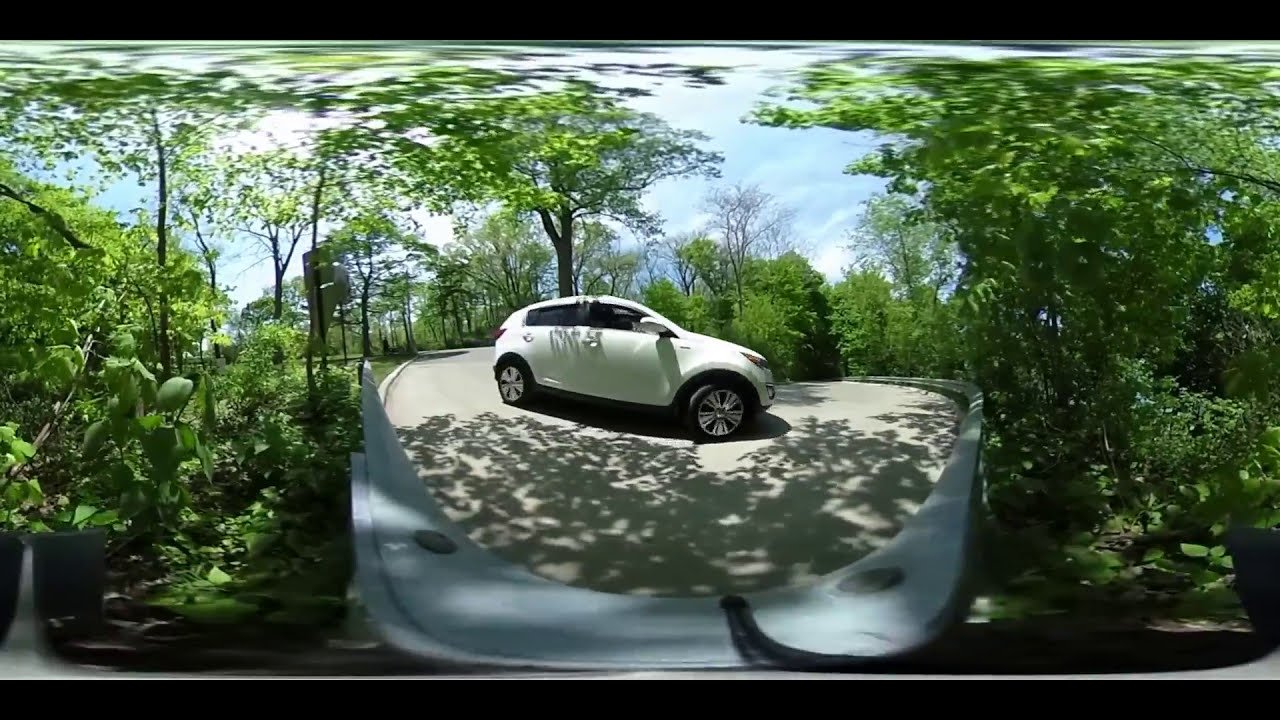The image captured through a fisheye lens shows a scene with some distortion, where objects appear rounded and slightly larger. The central focus is on a white SUV with metal rims featuring triangular designs and two slits inside them. This SUV is parked, its front wheel turned slightly to the left while the back wheel remains straight. Its lights are off, and a black roof rack can be seen on top of the vehicle.

The scene also includes a variety of greenery. Behind the SUV stands a singular tree topped with leaves, stretching towards a sky that is bright with a few clouds. To the right of the vehicle, there are numerous green bushes or smaller trees creating significant shade. Farther back, a leafless tree is visible, contrasting with the lush foliage around.

The area appears to be a dead-end road or a roundabout, marked by metal railings. Surrounding the scene are more trees, which due to the camera lens, look flattened at the top and somewhat blurred. These trees cast shadows on the image, adding to the natural environment pervasive throughout the scene. To the left and right, additional tall trees stretch upwards, contributing to a canopy-like effect. Green grass can also be seen underfoot, and there's an indistinct gray object protruding in front of the vehicle, adding some ambiguity to the setting.